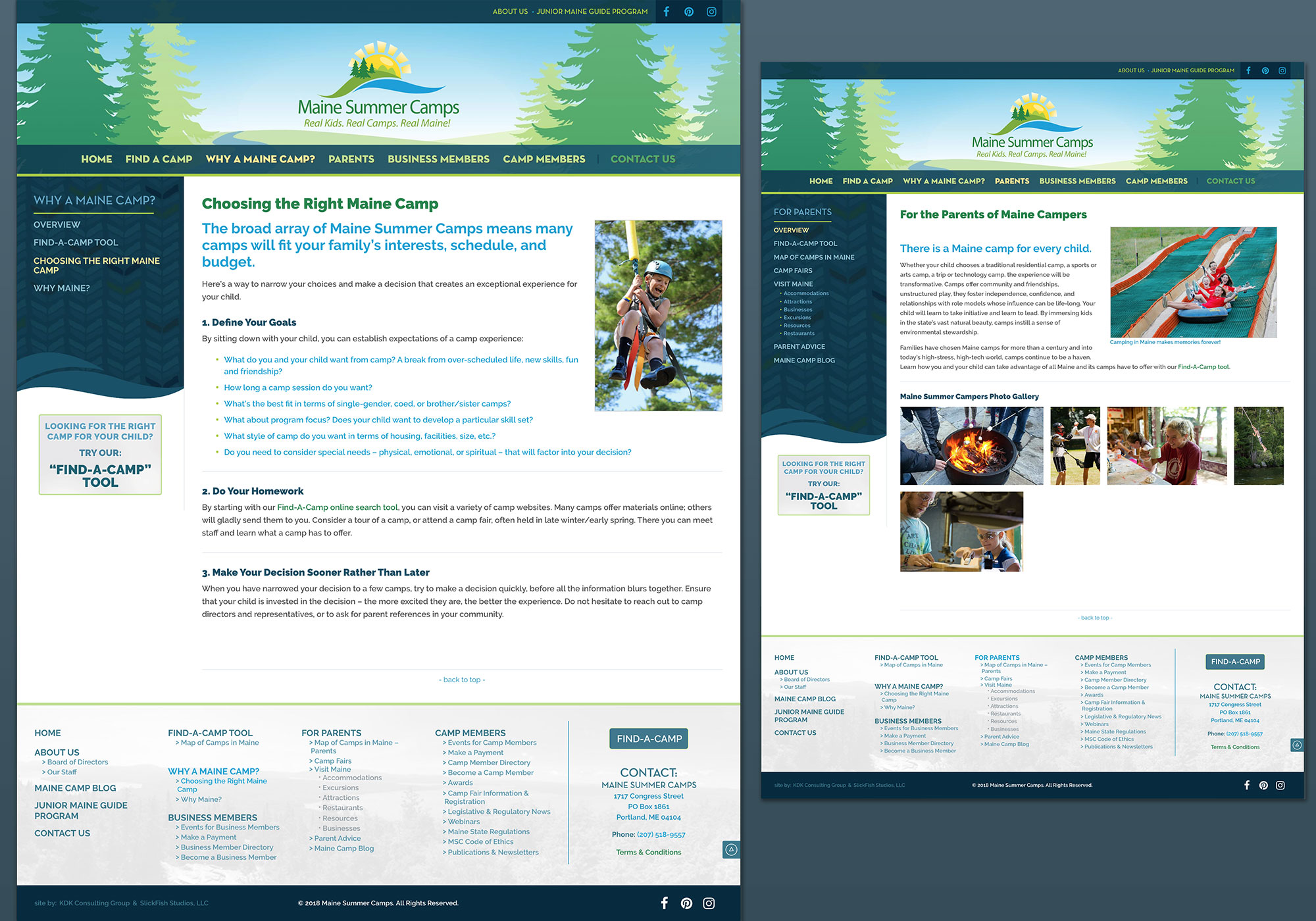**Maine Summer Camps: Fun, Friendship, and Adventure Await**

**Header Description:**
At the top, a computer-drawn border features lush green trees of various shades on either side, set against a blue sky. Between the trees, a field stretches out, traversed by either a river or a road, creating a picturesque scene. 

**Border and Navigation:**
The entire image is framed by a dark green border. Below the scenic header, the background shifts to a darker teal color. On a yellow strip, navigational links are prominently displayed in yellow text: "Home," "Find a Camp," "Why Maine Camp," "Parents," "Business Members," "Camp Members," and "Contact." These links help users navigate the website easily.

**Left Sidebar:**
On the left side, under the heading "Why Maine Camp," a green line separates the following sections: "Overview," "Find a Camp Tool," "Choosing the Right Maine Camp," and "Why Maine."

**Main Content Area:**
In the middle, on a clean white background, the text "Choose the Right Maine Camp" stands out. Below, in blue or green text, a detailed description guides families in selecting the perfect summer camp. 

"Maine's extensive array of summer camps means there are many options to fit your family's interests, schedule, and budget. Here’s how to narrow your choices and make a decision that creates an exceptional experience for your child:"

**Bullet Points:**
- **Define Your Goals:** Sit down with your child to establish what you both want from the camp experience. 
  - Break from over-scheduled life 
  - New skills 
  - Fun and friendships 
- **Camp Session Duration:** Decide on the length of the camp session.
- **Camp Type:** Choose the best fit based on single-gender, co-ed, or brother-sister camps.

This comprehensive breakdown ensures you select a camp that aligns perfectly with your family's needs and your child's aspirations.